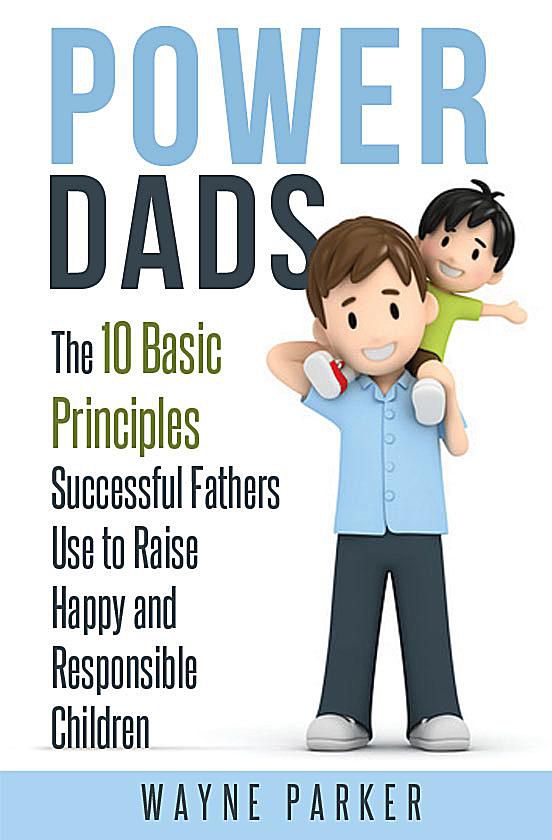The image appears to depict the cover of a book titled "Power Dads." At the top, "POWER" is written in large, light blue capital letters, followed by "DADS" in slightly smaller, darker blue letters. Below the title, in a left-hand column format, there is a heading that reads "The ten basic principles successful fathers use to raise happy and responsible children." Most of this text is in black, except for "ten basic principles," which is highlighted in green. On the right side of the cover, there's an illustration of a father with short brown hair wearing a light blue short-sleeved shirt, dark pants, and white shoes. He has a child on his shoulders, who has short black hair, wears a green shirt and dark pants, and is peeking out over the father's left shoulder with one hand extended to the side. At the bottom of the cover, there is a blue rectangle containing the author's name, Wayne Parker, written in black letters.